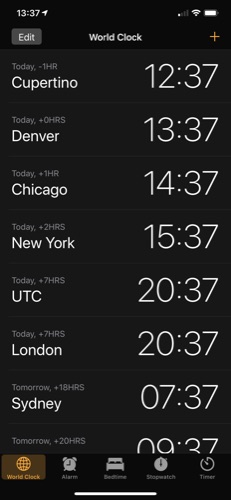The image captures a smartphone screen displaying the World Clock feature. At the top left corner, the local military time is 13:37 and an arrow icon indicates that location services are enabled. On the top right, icons for cell service, Wi-Fi, and battery status (without percentage) are visible.

Just below, the title "World Clock" is centered, flanked by a gray "Edit" button and an orange plus sign on the left and right, respectively, suggesting options to modify or add new clocks.

The main content lists several global cities with their current times:

- Cupertino shows 12:37
- Denver shows 13:37
- Chicago shows 14:37
- New York shows 15:37
- UTC shows 20:37
- London shows 20:37
- Sydney shows 07:37 the next day

The last city is partially cut off, but it appears to be 09:37. Above each city name, the time difference from the current location is noted in gray. For example, Cupertino is listed as "Today, -1 hour."

At the bottom, the World Clock tab is selected among other options like Alarm, Bedtime, Stopwatch, and Timer.